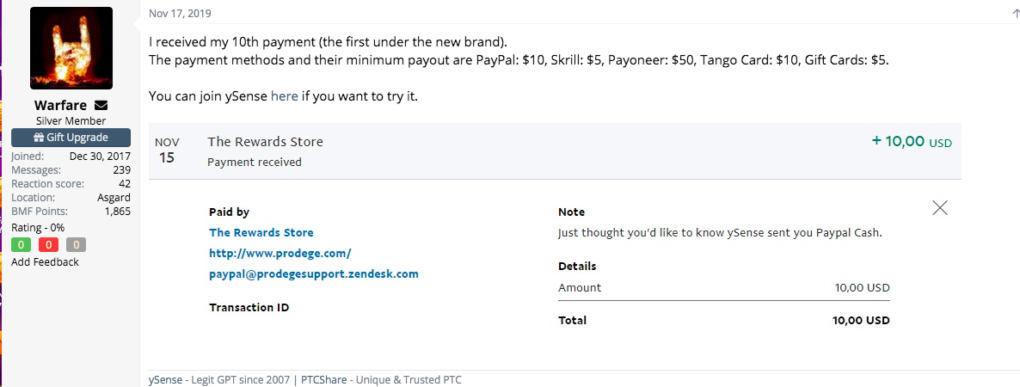**Detailed Descriptive Caption:**

This screenshot captures a payment screen interface, which is divided into two sections. On the left, there is a vertical gray panel featuring several elements. At the top of this panel, a user profile picture is displayed alongside a prominent box. Below the box, the text reads "Warfare" and "Username," followed by "Silver Member." Beneath this, there is a "Gift Upgrade" prompt accompanied by a blue button. Further down, the panel lists categories such as "Join," "Messages," "Reaction Score," "Location," "BMF Points," and "Rating." Adjacent to these categories are three colored boxes with zeroes in their centers— one green, one red, and one gray. At the bottom of the panel is an "Add Feedback" option.

To the right of the panel is a larger section with a white background. At the top, the date "November 17, 2019" is prominently displayed, followed by a user's comment. The comment states: "I received my 10th payment, the first one under the new brand. The payment methods and their minimum payout are PayPal, $10, Skrill $5, Payoneer $50, Tango Card $10, and Gift Cards $5. You can join YSense here if you want to try it," with the word "here" being hyperlinked. Below this comment, there is an embedded screenshot showing details of the payment received.